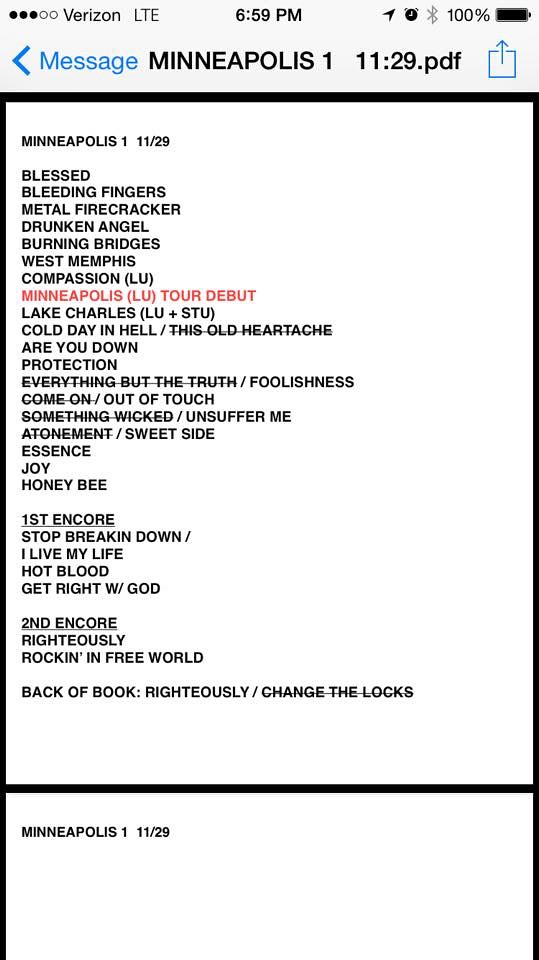The image is a screenshot from a phone displaying a PDF under the "Messaging" section. At the top, it reads "Minneapolis 1, 11/29." The document contains a detailed list of song titles written in black ink. The titles are:

"Blessed," "Bleeding Fingers," "Mild Firecracker," "Drunken Angel," "Burning Bridges," "West Memphis," "Compassion," followed by "Minneapolis LU Tour Debut" in red ink, then "Charles LU + STU," "Cold Day in Hell," "This Old Heartache" (crossed out), "Are You Down," "Protection," "Everything But The Truth" (crossed out), "Foolishness," "Come On," "Outta Touch," "Something Wicked," "Unsuffer Me," "Atonement," "Sweet Side," "Essence," "Joy," and "Honey Bee." 

The next segment, underlined and labeled "First Encore," lists "Stop Breaking Down," "I Live My Life," "Hot Blood," and "Get Right With God." Another segment labeled "Second Encore" includes "Righteously" and "Rockin' In The Free World." Finally, the list ends with "Back of Book Righteously Changes The Locks."

The background is predominantly white with the titles in black and one segment in red. The phone's typical menu icons and the current time are visible at the top of the screenshot. This appears to be a setlist for a musical performance.